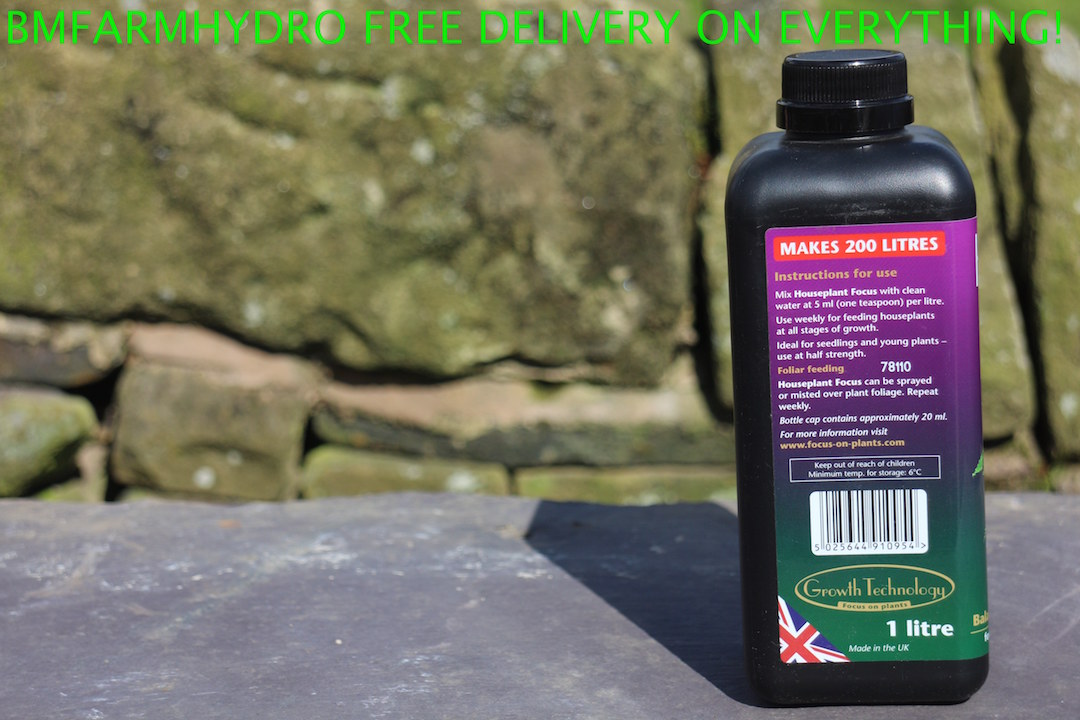The photograph features a black plastic bottle, likely containing plant food or a plant growth enhancer, positioned on a gray stone outdoors, with a green-tinted stone wall in the background. The bottle, capped in black, is adorned with a label that transitions from purple at the top to green at the bottom. Prominently displayed on the label are the phrases "makes 200 liters" and "instructions for use." At the top of the image, in bold green capital letters, it reads, "BM Farm Hydro, free delivery on everything." The label includes additional details, such as a British flag in the lower left corner, a barcode, the words "growth technology," "one liter," and "made in the UK." The bottle's label also provides instructions specifically tailored for houseplant care, a website in orange, a warning to keep out of reach of children, and the manufacturer's logo.